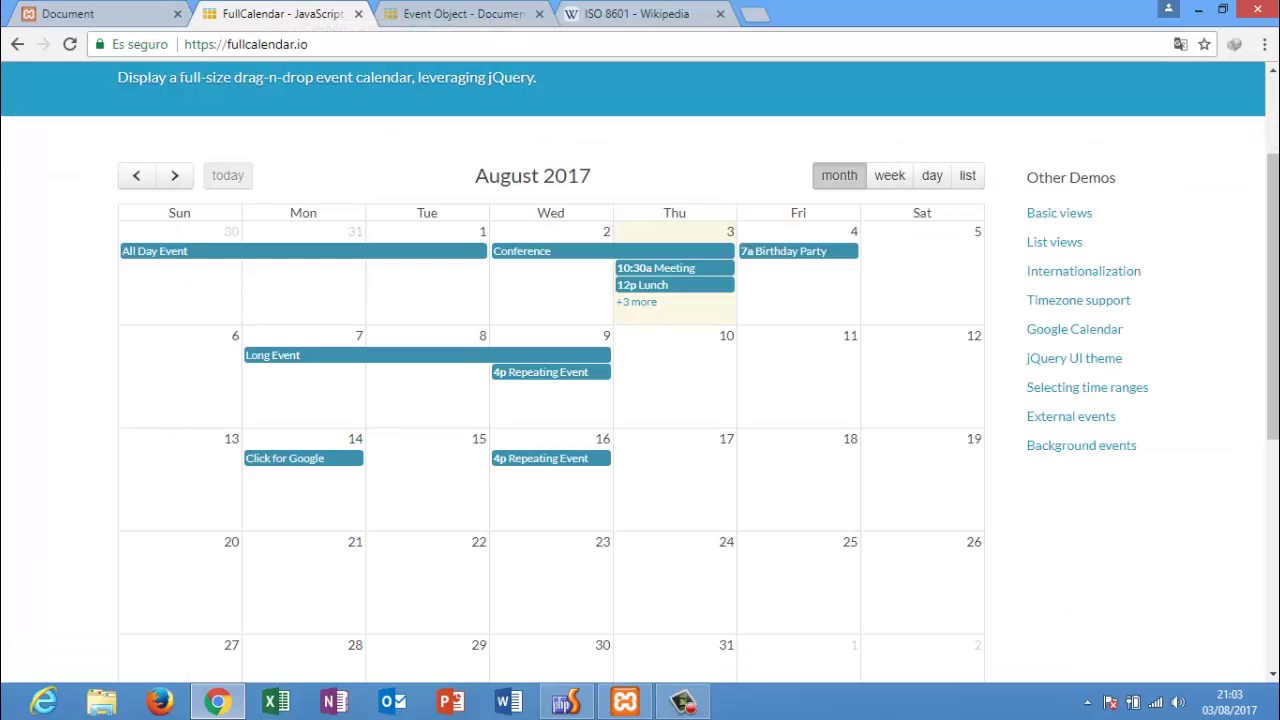The image is a screenshot of a maximized Microsoft Edge browser window on a Windows desktop. The browser has four open tabs, with the active tab displaying the "FullCalendar JavaScript" page from the URL "https://fullcalendar.io". This tab shows a calendar for August 2017, featuring several meetings and all-day events highlighted in blue.

Besides this, the other three tabs are:
1. A document tab.
2. An event object-document tab.
3. A Wikipedia entry for ISO 8501.

At the bottom of the desktop, the taskbar includes icons for Internet Explorer, Firefox, Chrome, File Explorer, and various Microsoft Office applications. Additionally, there are a few unfamiliar icons: an orange 'S' and an orange and white dog bone icon. The date and time displayed on the taskbar are March 13, 2017, at 10:03 PM.